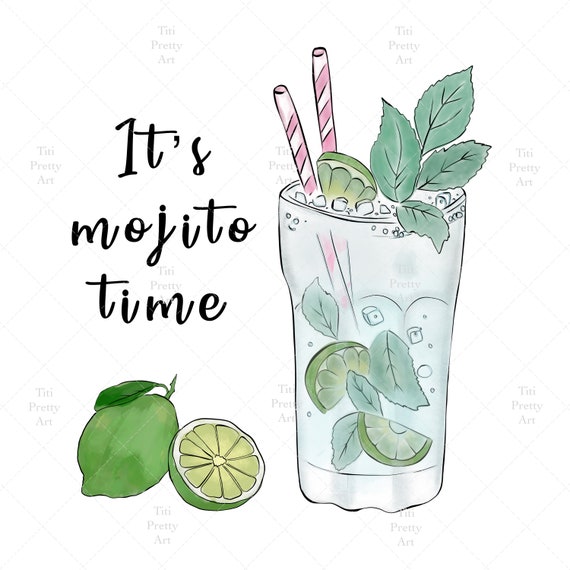The image is a detailed and vibrant depiction of a refreshing mojito drink, set against a clean white background adorned with a light blue or gray crisscross diamond pattern. Within every third diamond, subtle light gray text reads "T.I.T.I Pretty Art," serving as a watermark. Central to the image, slightly toward the right, stands a large glass of mojito, tinted with a hint of blue. The glass contains ice cubes, slices of lime, and mint leaves, topped with more mint and a slice of lime. Two red and white diagonal striped straws protrude from the beverage, enhancing its lively appearance. To the left of the glass, in bold black print, the text proclaims, “It’s mojito time.” Below this text, there is a whole green lime with a leaf attached at its stem, and beside it, a halved lime revealing its juicy interior. The colors are predominantly green, yellow, and the distinct red and white of the straws, all contributing to the bright and fresh feel of the image. The entire setting is bathed in natural light, giving it a clear and bright atmosphere.